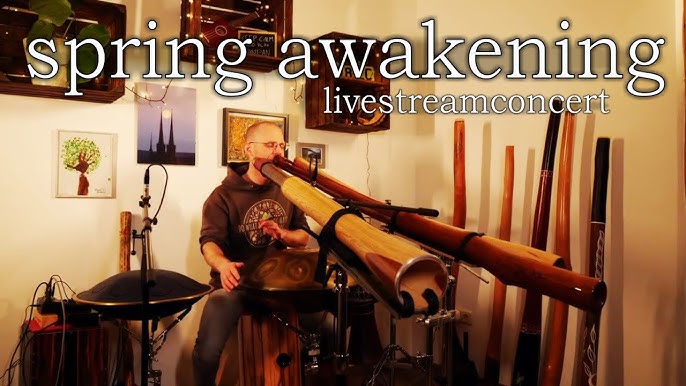In the image, a man sits on a wooden stool in a room with white walls adorned with various pictures and shadow boxes filled with random items. He wears glasses, a black hoodie with a design on the front, and jeans, and appears to be bald. In front of him are three long, hollow wooden pipes, likely musical instruments, with the central one being longer and secured by brackets. To his left, there's a cymbal or a similar percussion metal instrument, while on his right is a black hand drum. Additional wooden pipes of different colors lean against the right-hand wall. Above the man, white text reads "Spring Awakening Livestream Concert," indicating that he is performing at a live stream event.